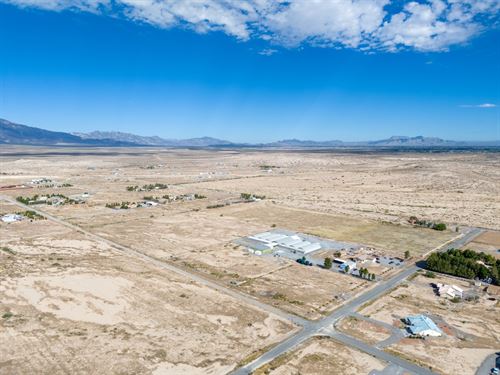This aerial photograph captures a predominantly barren, desert landscape with a sweeping horizon crowned by distant mountains. The sky transitions from a dark blue at the top to lighter blue near the horizon, punctuated by bright white clouds and illuminated by sunlight. Dominating the main body of the image is a vast expanse of sandy, tan-colored land, sparsely dotted with green vegetation. Situated in the foreground is a complex consisting of a gray parking lot with white structures, flanked by green pine trees. Nearby, an intersection of two roads is visible, creating a grid pattern that defines the area. Along one side of the intersection lies a large house with surrounding acreage, perhaps used for businesses such as landscaping, indicated by the presence of greenhouses. Across the road, a dense cluster of tall green trees hides another house. Despite a few isolated properties and scattered trees, the majority of this expanse remains open desert, hinting at either a rural or a developing residential area.